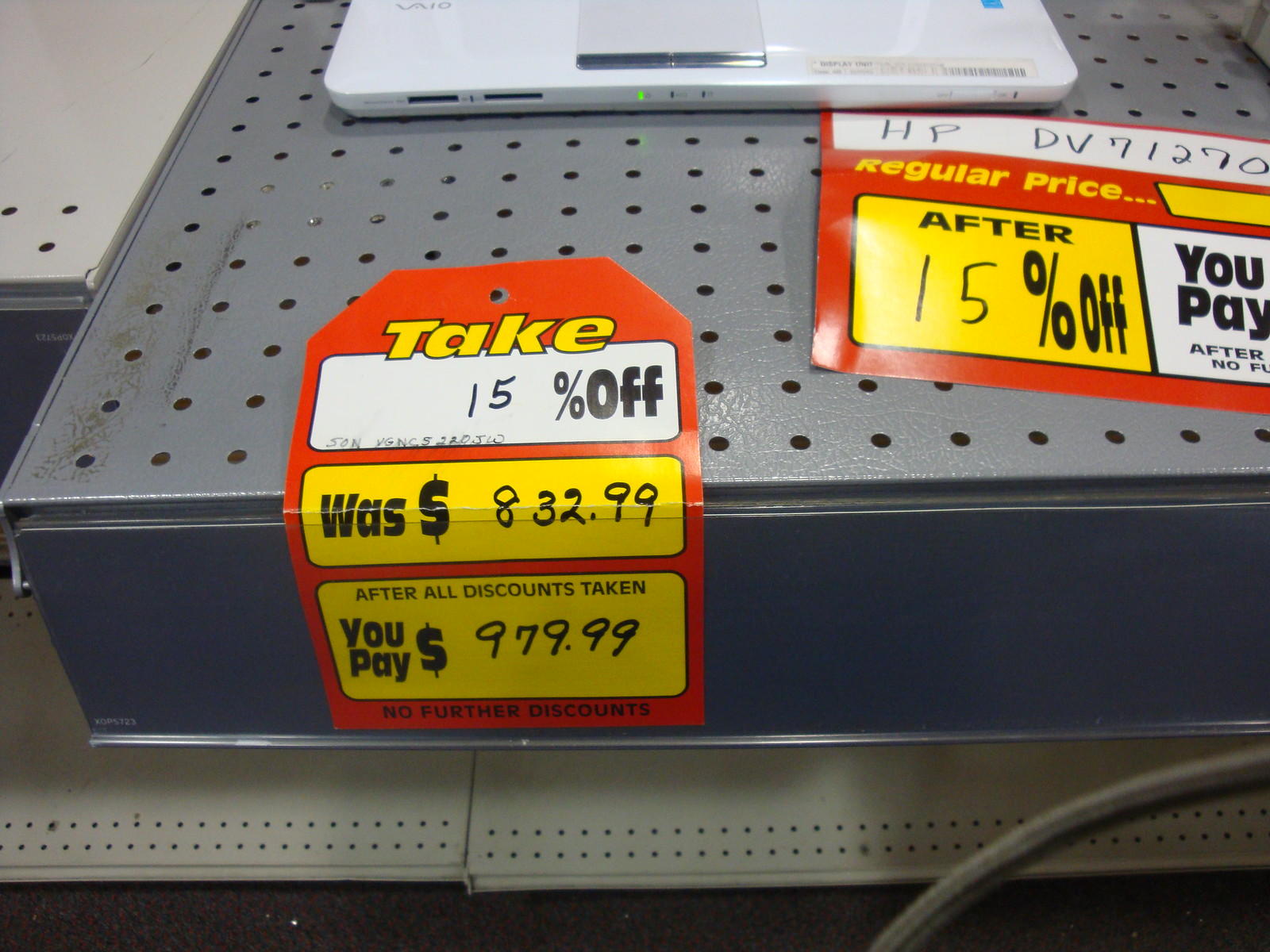This photograph captures an interior view of a store display, focusing on a close-up of metal gray perforated racks adorned with sample electronics. Prominently featured at the top of the image is a white laptop, of which only the bottom edge and the mouse pad are visible. On the left side of the frame, closer to the bottom, a large red sticker stands out. The sticker reads: "Take 15% off, was $832.99, after all discounts taken, you pay $979.99. No further discounts." To the right, another price sticker shows a partial label that reads: "HPDV 171270. After 15% off, you pay," with the rest of the text obscured. The overall scene suggests a sale or promotional setup for electronic devices in the store.